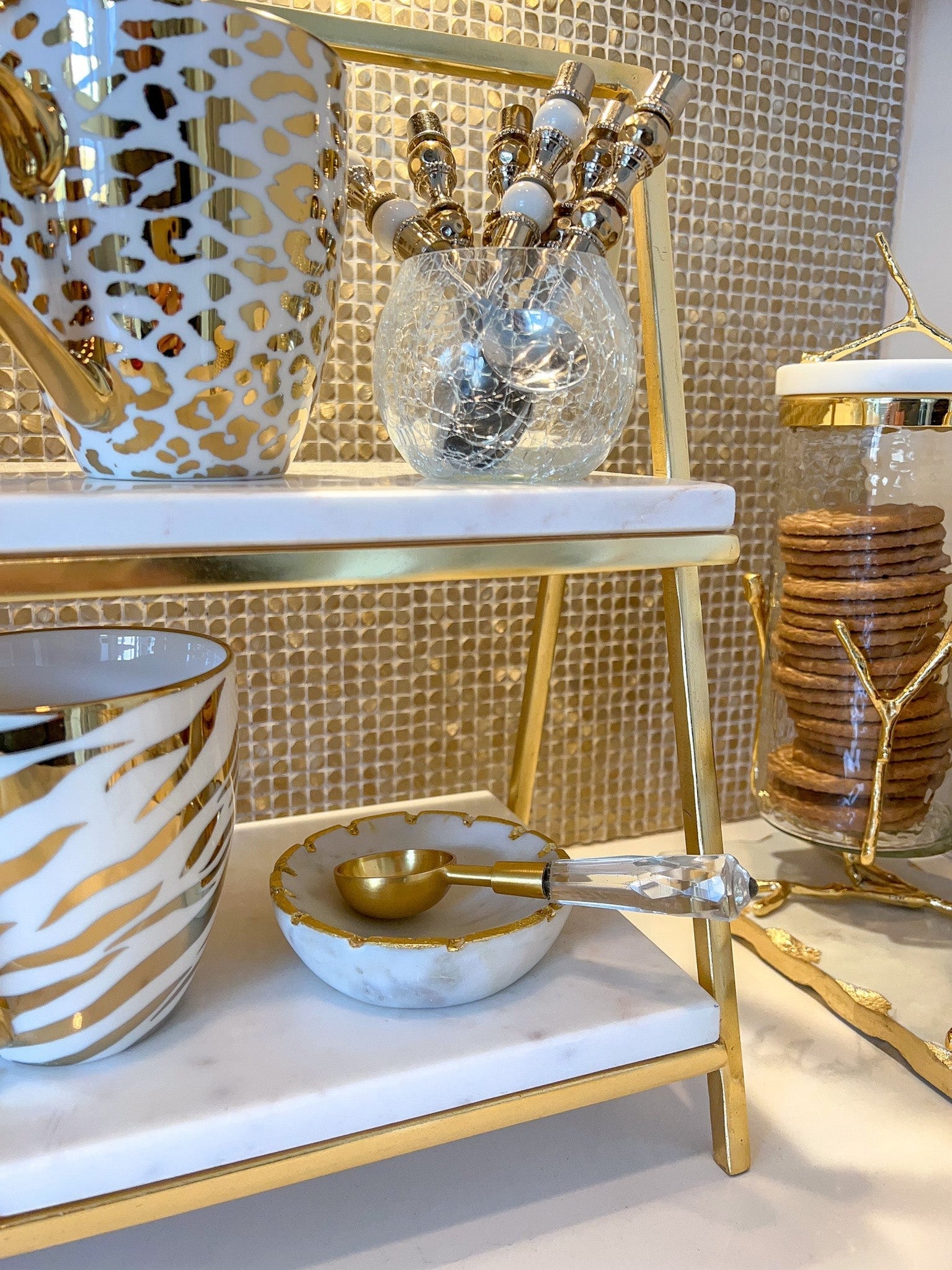The image depicts a lavish and meticulously organized coffee and tea station, set against an opulent gold mosaic backsplash. Dominating the left side is an elegant two-tiered stand with marble shelves supported by brass fittings. On the top tier, a striking white coffee mug adorned with cheetah-patterned gold accents sits next to an old-fashioned crackled glass holding an assortment of decorative spoons with gold and white handles. The bottom tier houses another exquisite mug, this time featuring a zebra pattern in gold on a white background, and a white marble dish that holds a gold coffee scoop with a lucite handle. To the right, a glass cookie jar with a white marble top and subtle gold accents contains neatly stacked golden cookies, adding a touch of homely charm to this luxurious setup. The entire scene is set on a pristine white marble kitchen counter, enhancing the station's sophisticated aesthetic.